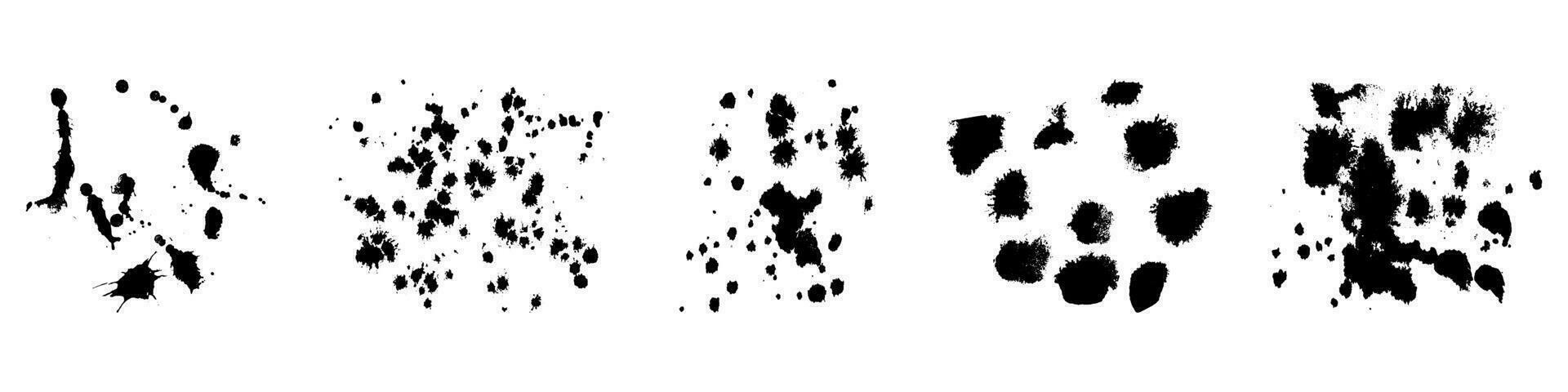The image displays a series of five distinct patterns of black ink splotches arrayed horizontally across an elongated white background. On the far left, the first pattern showcases a chaotic mix of variously sized ink splotches, ranging from large to small, dispersed without any recognizable design. To the immediate right, the second pattern features a dense arrangement of very small, evenly-sized black specks, resembling a concentrated spray. The third pattern continues with small ink splotches interspersed with larger ones, creating a more filled and complex design. Moving further right, the fourth pattern consists exclusively of substantial, fuzzy-edged ink splotches, arranged in a circular yet squarish configuration. Finally, the far-right pattern displays an array of very large, indistinct black blobs intermixed with smaller splotches, creating a juxtaposition of sizes and intensities.